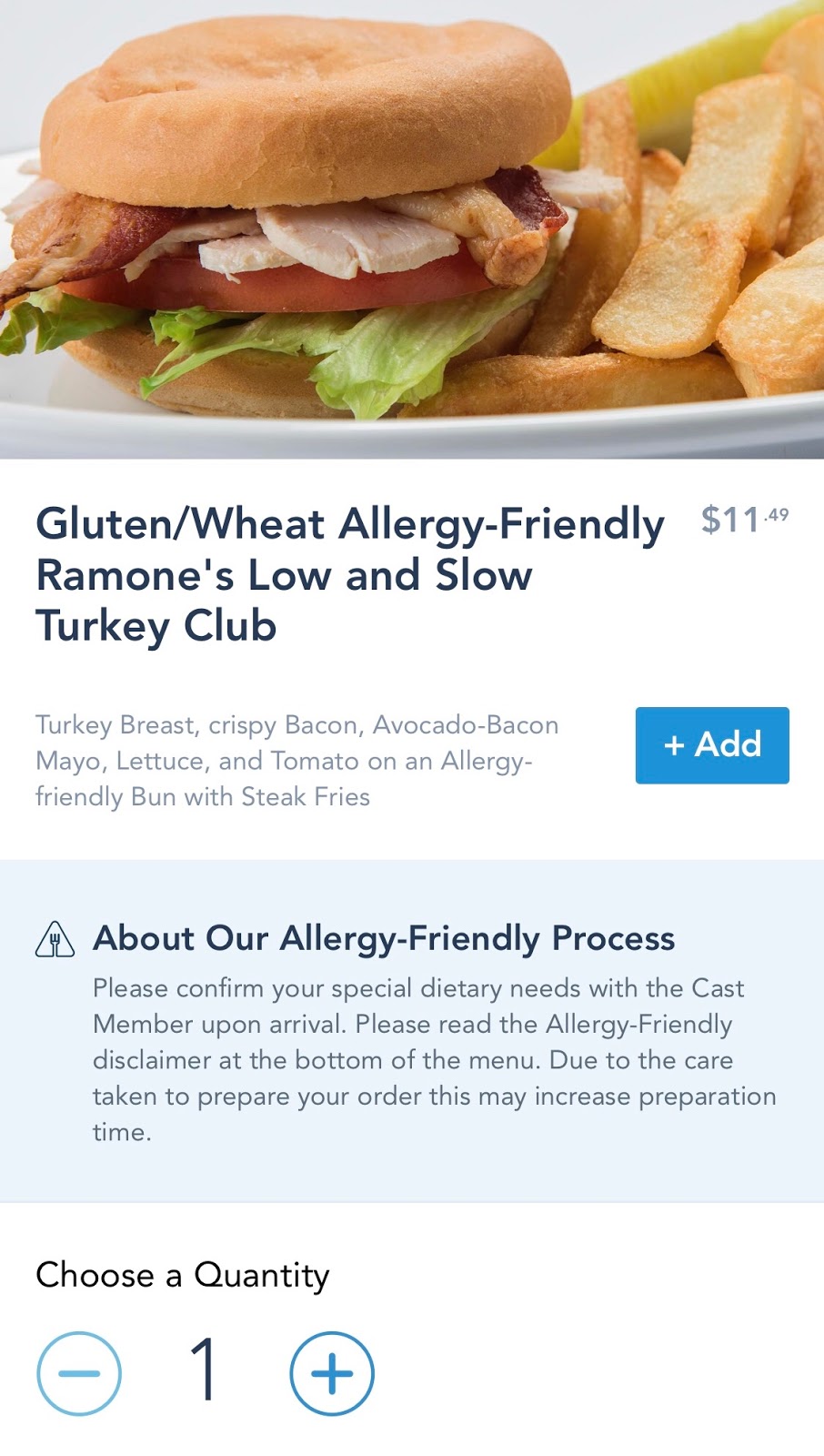This image features an advertisement for a sandwich at Ramone's. At the top, a delectable turkey club sandwich is prominently displayed. The sandwich includes juicy turkey, crispy bacon, creamy avocado, fresh green lettuce, and bright red tomato, all nestled between slices of an allergy-friendly bun. Accompanying this mouth-watering sandwich are golden, crisp steak fries, all beautifully presented on a white plate. A pickle peeks out from the background, adding a final touch to the appetizing presentation.

Below the image, text highlights the sandwich’s name and features: "Ramone's Low and Slow Turkey Club." It specifies this option as gluten and wheat allergy-friendly. Detailed in smaller letters are the ingredients: turkey breast, crispy bacon, avocado, bacon mayo, lettuce, and tomato, served on an allergy-friendly bun with steak fries.

A blue rectangle with the text "Plus Add" indicates an option to add the item to your cart, priced at $11.49. A larger light blue rectangle below that explains Ramone's allergy-friendly process, advising customers to confirm special dietary needs with a cast member upon arrival and to read the allergy-friendly disclaimer at the bottom of the menu. It also notes that the care taken in preparation may increase preparation time.

At the bottom, options are provided to choose a quantity, with a minus and plus sign flanking a number one.